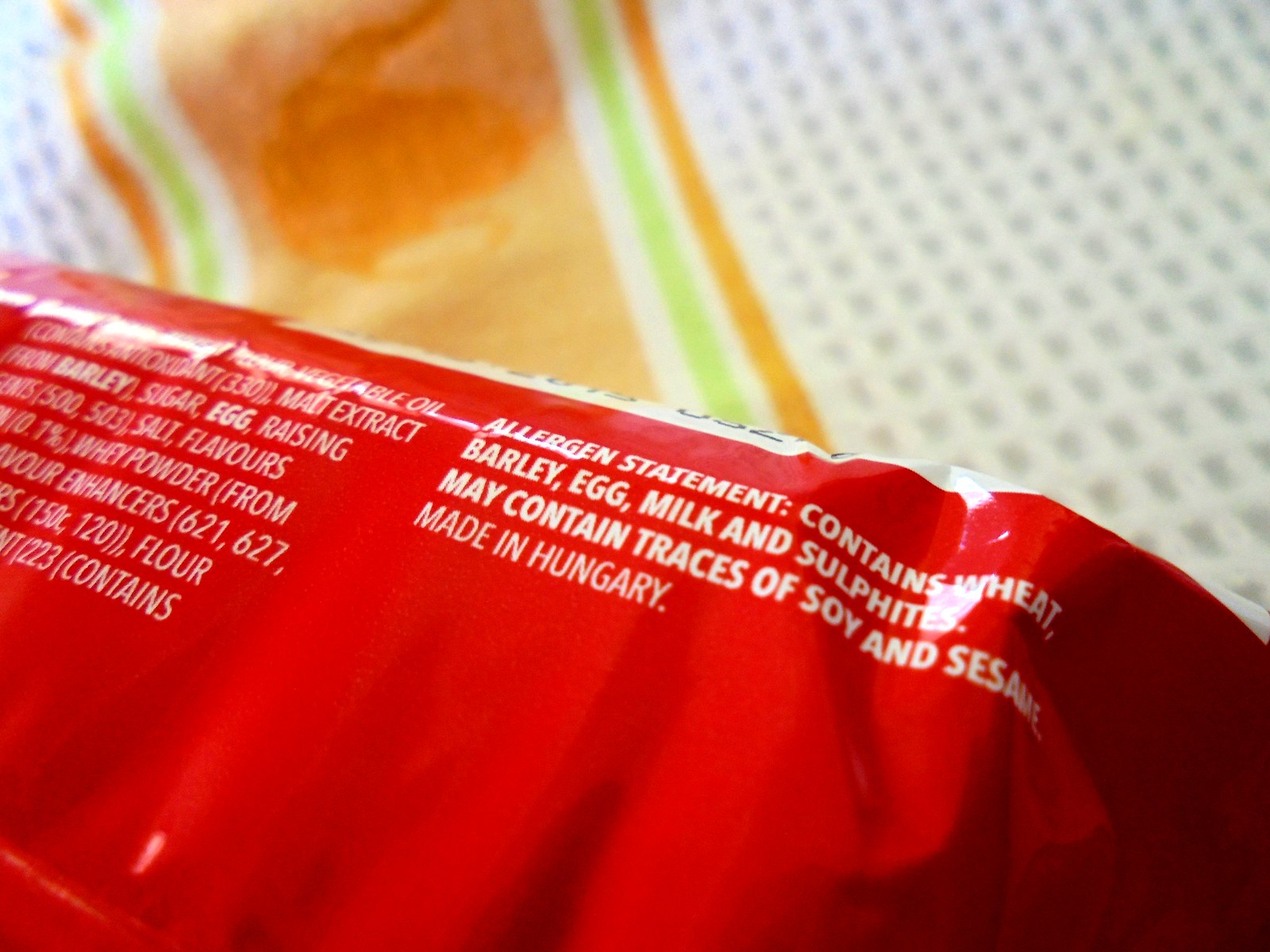This is a close-up photograph of a long, red package of food, which appears to be made of a plastic material commonly seen in frozen food sections. The package prominently displays a white allergen statement, indicating it contains wheat, barley, egg, milk, and sulfites, and may contain traces of soy and sesame. Additionally, it mentions that the product is made in Hungary. The image shows some additional text and ingredients such as malt extract, barley, whey powder, and flour, although much of this text is obscured by glare. The background consists of a casual, colorful tablecloth with white, orange, and lime stripes.